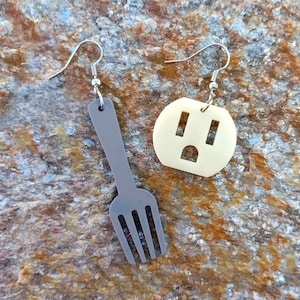The photograph showcases a pair of avant-garde earrings set against a background resembling a rock or mineral surface with hues of white, gray, silver, blue, and copper tones. The first earring takes the form of a gray plastic fork, featuring four prongs and a simplistic, almost cartoonish design. Its silver hook, designed for ear piercing, attaches through a hole at the top of the fork. The second earring mimics a white electrical outlet cover, bearing a hexagonal shape reminiscent of a stop sign, with two rectangular "eyes" and a U-shaped "mouth," resembling the face of a typical socket. The earrings appear together as a whimsical and humorous commentary on the hazards of inserting forks into electrical outlets.